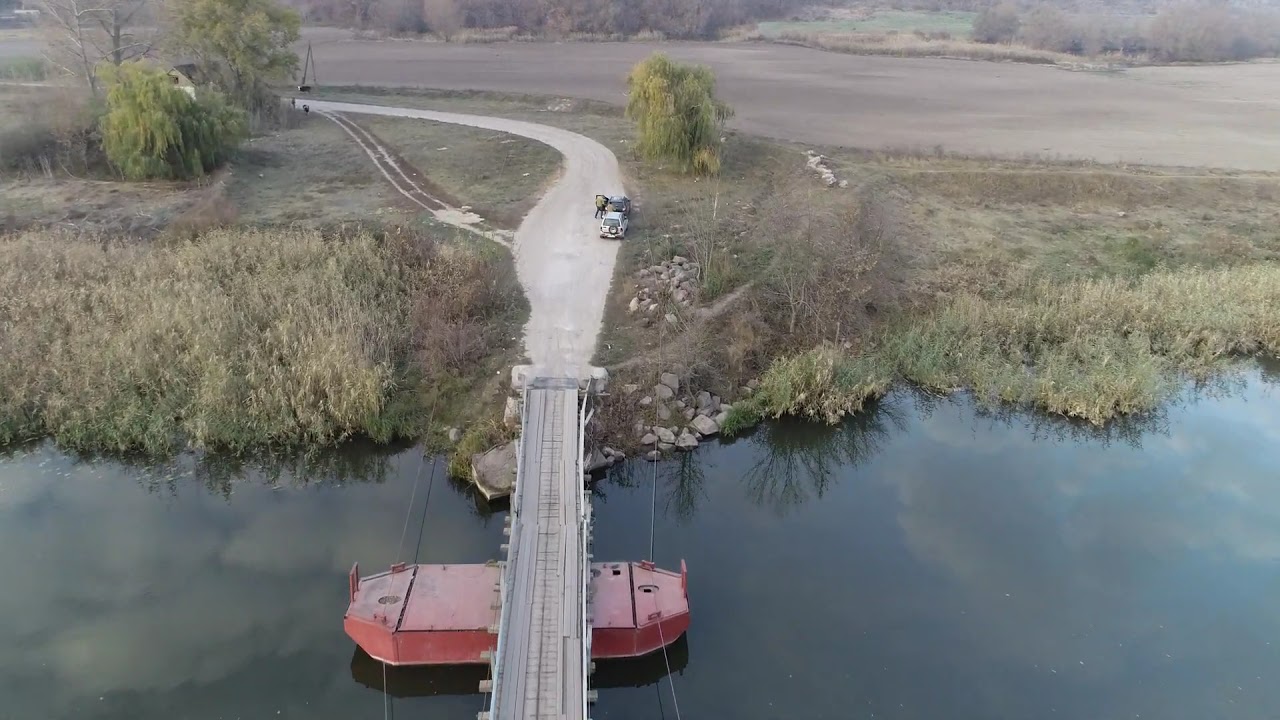The image features a serene rural scene dominated by a still pond in the foreground, reflecting the light blue sky and clouds above. A single-lane gray bridge, appearing somewhat crude and makeshift, spans the pond. The bridge is supported by a large, red, raft-like structure beneath it. Extending from the bridge is a gravel road leading up and to the left, with a truck parked near its starting point and another white car further along the path. A person stands beside one of the vehicles. To the right of the truck, there is a cleared area with visible vehicle tracks. Surrounding the scene, green brush lines the pond's edge transitioning to dry, brown plains in the background, accentuated by three weeping willow trees. A small house with part of its roof visible is nestled in the distance. The color palette of the image includes light greens, browns, and grays, adding to the rustic, tranquil atmosphere. There is no text in the image.